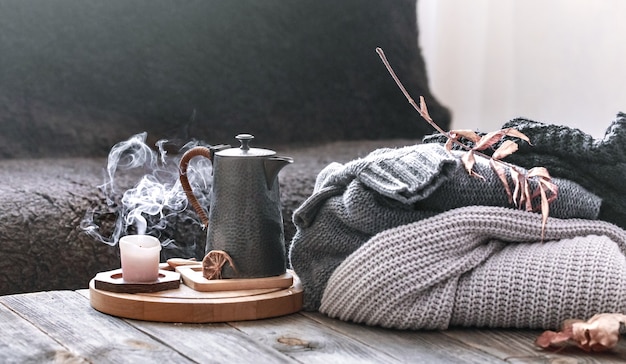In this picture, we see a wooden table with diagonal white and gray slats. On the table is a round wooden tray that holds various items. The tray features a gray teapot with brown handles, positioned on a wooden saucer. Beside the teapot sits a recently extinguished candle, its wick still releasing a trail of white smoke. The candle is purple-red in color. Adjacent to the tray, there is a bundle of clothing comprising thick, woolen sweaters in shades of gray, black, and brown. A few withered fall leaves are scattered on and around the clothes, emphasizing the end of summer. In the background, we observe a gray sofa with fluffy gray cushions, and to the right side of the image, a white curtain. The overall scene gives off a cozy, autumnal vibe filled with rustic and homely elements.